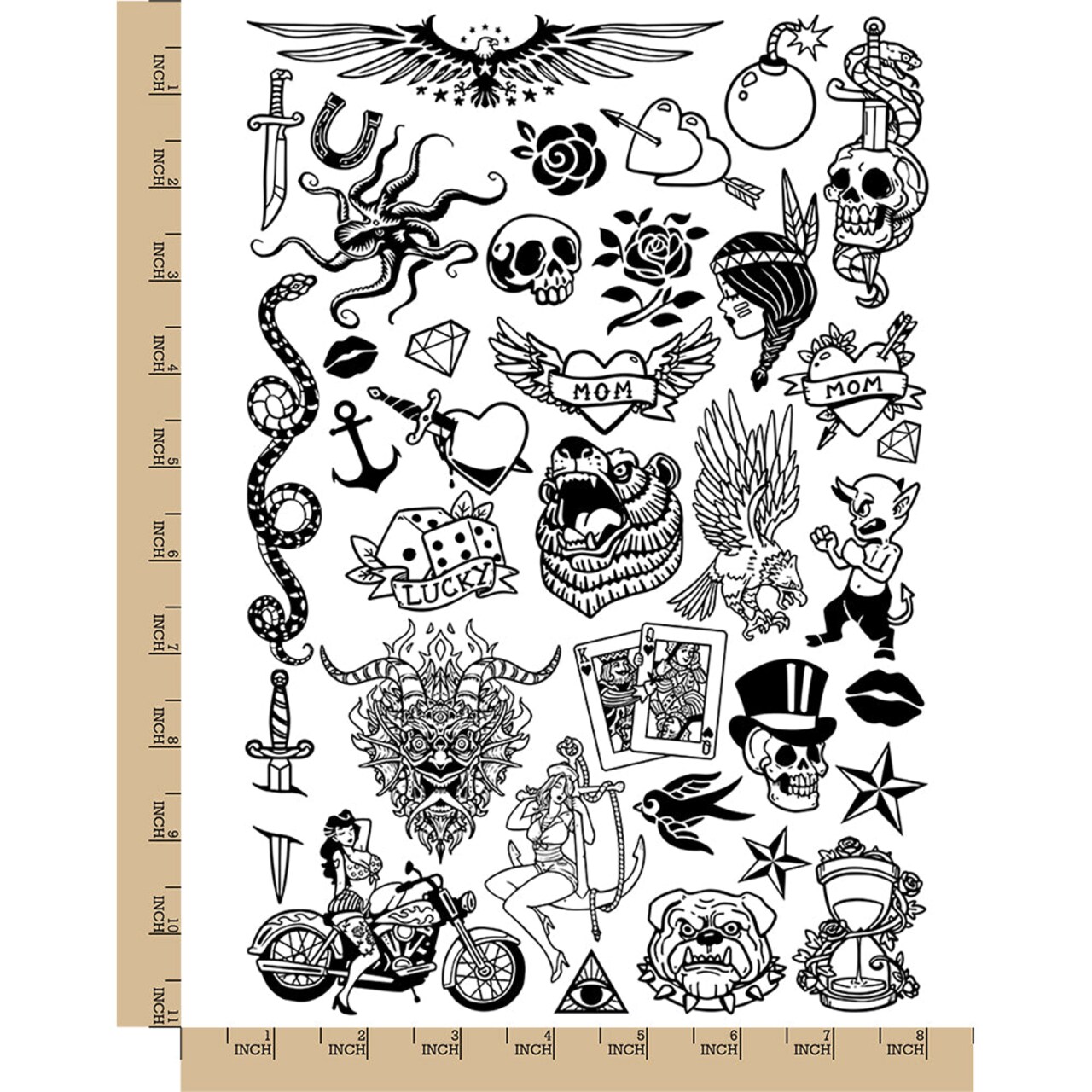The image appears to be a collection of hand-drawn tattoo stencil designs arranged along the left side and bottom of a white background, possibly a notebook cover. These black and white illustrations include a wide variety of typical tattoo motifs. For instance, there is a heart with wings that says "mom" in the center, a detailed skull with a sword pierced through it and a snake coiled around the blade, and an anchor symbol. Other designs feature a woman on a motorcycle, a woman on an anchor, and a stern-looking bear head. Additional iconic imagery includes black lips, a heart with a dagger through it, an all-seeing eye inside a pyramid, a playing card set of a king and queen, a Native American woman with leaves in her hair, and several renditions of eagles, stars, and birds. At the bottom of the image runs a scale from 1 inch to 8.5 inches, while the left side features a similar ruler ranging from 1 inch to 11 inches, providing a sense of the actual size of these detailed stencil templates.